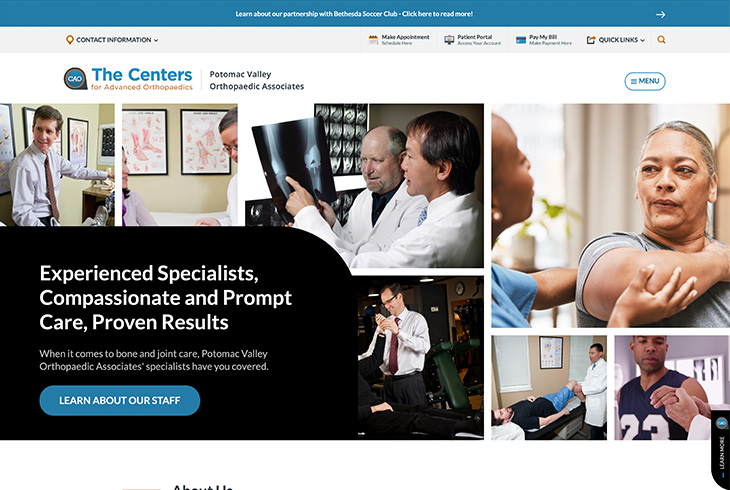The image depicts the homepage of the Centers for Advanced Orthopedics, Potomac Valley Orthopedic Associates. In the top left corner, there is clickable contact information. The top menu bar includes options for "Make an Appointment," "Patient Portal," "Pay My Bill," and "Quick Links." A prominent blue banner announces a partnership with the Bethesda Soccer Club, inviting users to "Click here to read more."

The main section of the page highlights their focus on x-rays and consultations, with captions emphasizing "Experienced Specialists," "Compassionate and Prompt Care," and "Proven Results." It states, "When it comes to bone and joint care, Potomac Valley Orthopedic Associates specialists have you covered. Learn about our staff."

On the right-hand side, imagery shows a patient receiving physical therapy on their arm, while other images below depict patients undergoing rehabilitation exercises for their leg and hand, respectively. The left-hand side prominently features information about the doctors and their services, emphasizing the comprehensive care provided for muscle and joint rehabilitation.